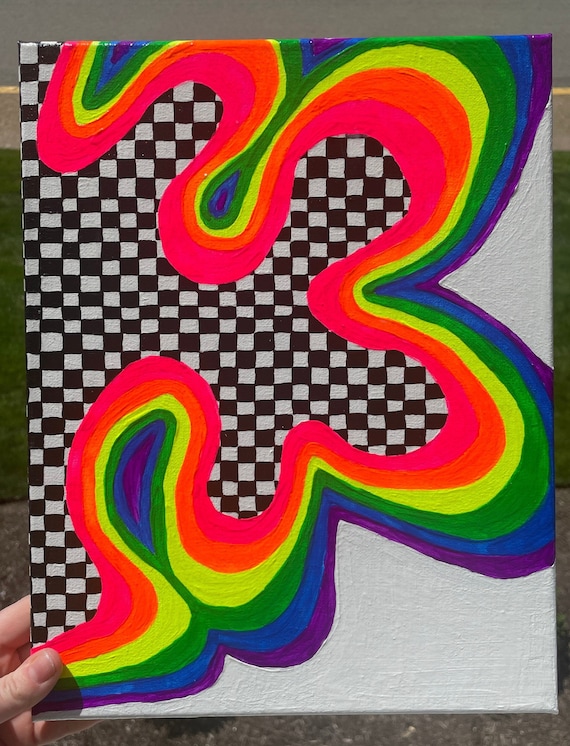The image depicts a vibrant, modern artwork, likely an oil painting on a small canvas, being held up by a hand—visible in the bottom left corner, showing a Caucasian thumb and forefinger. The painting features a captivating swirl of rainbow colors—red, orange, yellow, green, blue, and purple—starting from the upper left corner, swirling around the canvas in dynamic, roller coaster-like loops. This colorful swirl encloses a bold, black and white checkerboard pattern, reminiscent of checkered van shoes. The canvas itself has an off-white background, peeking through at the edges. The environment in the background suggests an indoor setting, with a bit of a wall and gray flooring visible. The painting appears to be showcased for appreciation rather than for sale, highlighting the artist's vivid and intricate design.